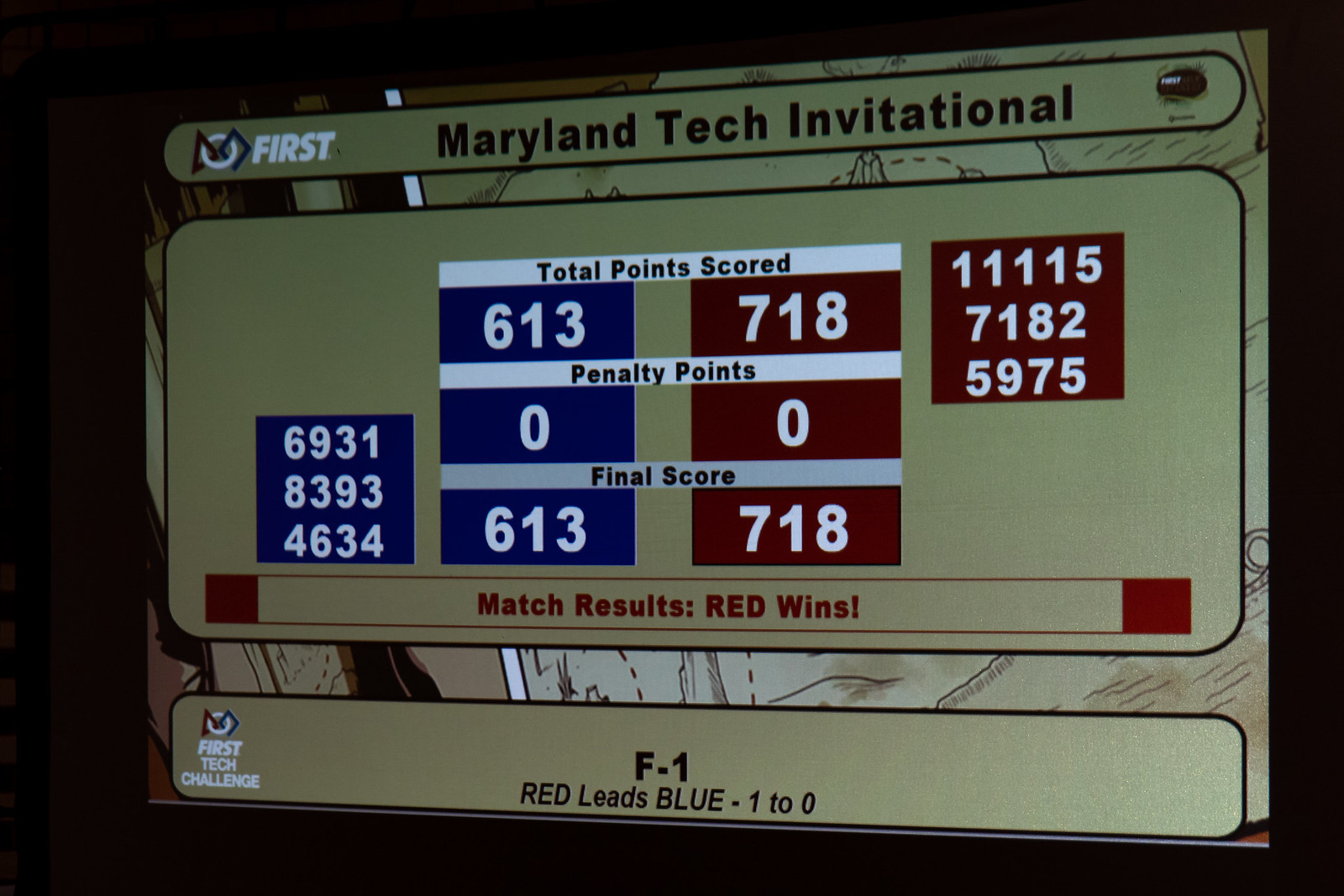This image features a close-up view of a detailed scoreboard set against a black background. The scoreboard itself is predominantly olive green with some cream-colored sections. At the very top, "Maryland Tech Invitational" is prominently displayed, accompanied by a football logo on the right. Beneath this heading lies the main scoreboard panel, segmented into various sections for clarity. The first row lists the total points scored, showing 613 for the blue team on the left and 718 for the red team on the right. Penalty points are evenly matched at 0-0. Following this, the final scores are reiterated, with the blue team at 613 and the red team at 718. 

There are two additional columns displaying expansive numeric data against colored backgrounds: the blue team's numbers (693, 183, 934, 634) and the red team's numbers (1111, 1571, 825, 975), adding to the granularity of the score tracking. The bottom section declares the match result, stating "Red wins" and further detailing that 'F1 red leads blue 1-0.' The comprehensive layout and distinct color coordination between blue and red for different teams highlight the competitive nature of the event.